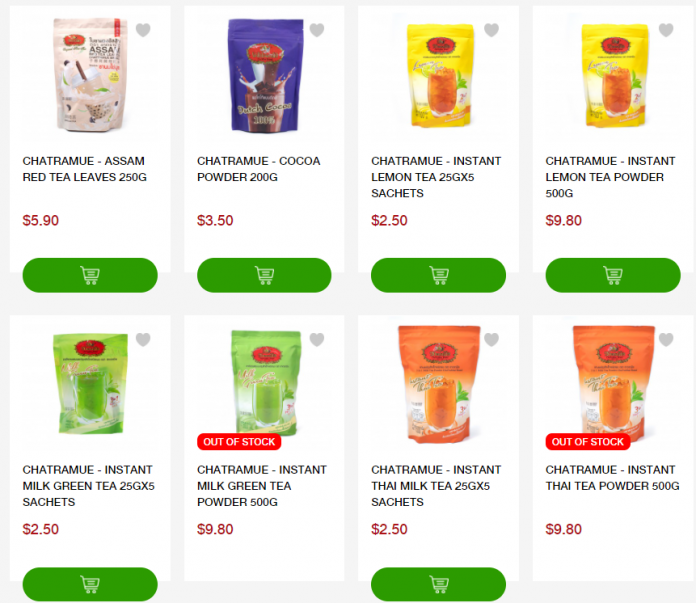A vibrant color image from an unidentified website displays a variety of tea products lined up in two rows. In the top row, from left to right:

- A light brown bag labeled "Chatramue Assam Red Tea Weaves," weighing 250 grams and priced at $5.90.
- A dark blue packet labeled "Chatramue Cocoa Powder," weighing 200 grams and priced at $3.50.
- A yellow packet labeled "Chat Ramieux Instant Lemon Tea," containing 25 grams per sachet, 5 sachets in total, priced at $2.50.
- Another yellow packet labeled "Chat Ramieux Instant Lemon Tea Powder," weighing 500 grams and priced at $9.80.

In the second row, from left to right:

- A green packet labeled "Chat Ramieux Instant Milk Green Tea," containing 25 grams per sachet, 5 sachets in total, and priced at $2.50.
- A green bag with a red "Out of Stock" banner, labeled "Chat Ramieux Instant Milk Green Tea Powder," weighing 500 grams and priced at $9.80.
- A brown bag labeled "Chat Ramieux Instant Thai Milk Tea," containing 25 grams per sachet, 5 sachets in total, priced at $2.50.
- An orange bag with a red "Out of Stock" banner, labeled "Chat Ramieux Instant Thai Tea Powder," weighing 500 grams and priced at $9.80.

The diverse array of tea products offers a comprehensive selection ranging from instant teas in various flavors to cocoa powder.